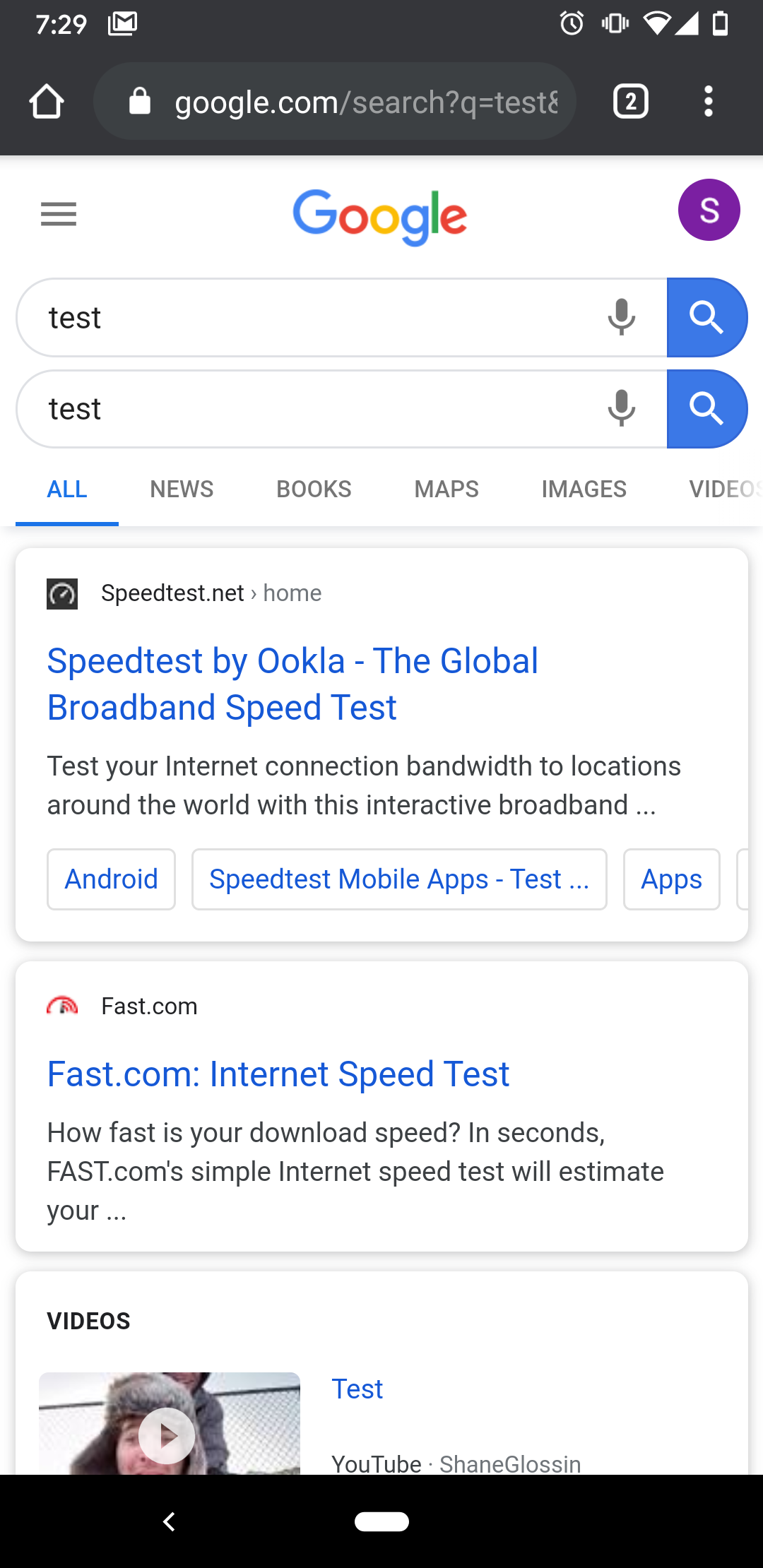The image captures a cluttered mobile dashboard on an Android device with several icons and a busy browser interface. Visible on the status bar are the Gmail icon, alarm, vibrate mode, Wi-Fi, and mobile data icons. The battery icon indicates it is nearly depleted. A home button and a white padlock icon are present on the screen.

In the browser, the URL displayed is "google.com/search?q=test" accompanied by a white search box with the digit '2' and three white dots indicative of loading or pagination, along with a menu icon showing three gray lines. Google’s logo is prominently displayed next to an 'S' character, with options for voice search. Various Google search tabs are available like All, News, Books, Maps, Images, Videos.

The web page currently opened appears to be detailing 'speedtest.net' by Ookla, highlighting its use as a global broadband speed testing service with the tagline "Test your internet connection bandwidth to locations around the world with this interactive broadband." Additionally, there are mentions of related mobile apps for Android and services like fast.com—a simple internet speed test tool by Netflix—as well as other terms like "YouTube."

Adjacent to this busy interface is an image of Shane Glosson, recognizable by the back arrow and a white dot against a black background. The thumbnail features a man wearing a fur hat with a play button superimposed over his face, suggesting a video ready for playback.